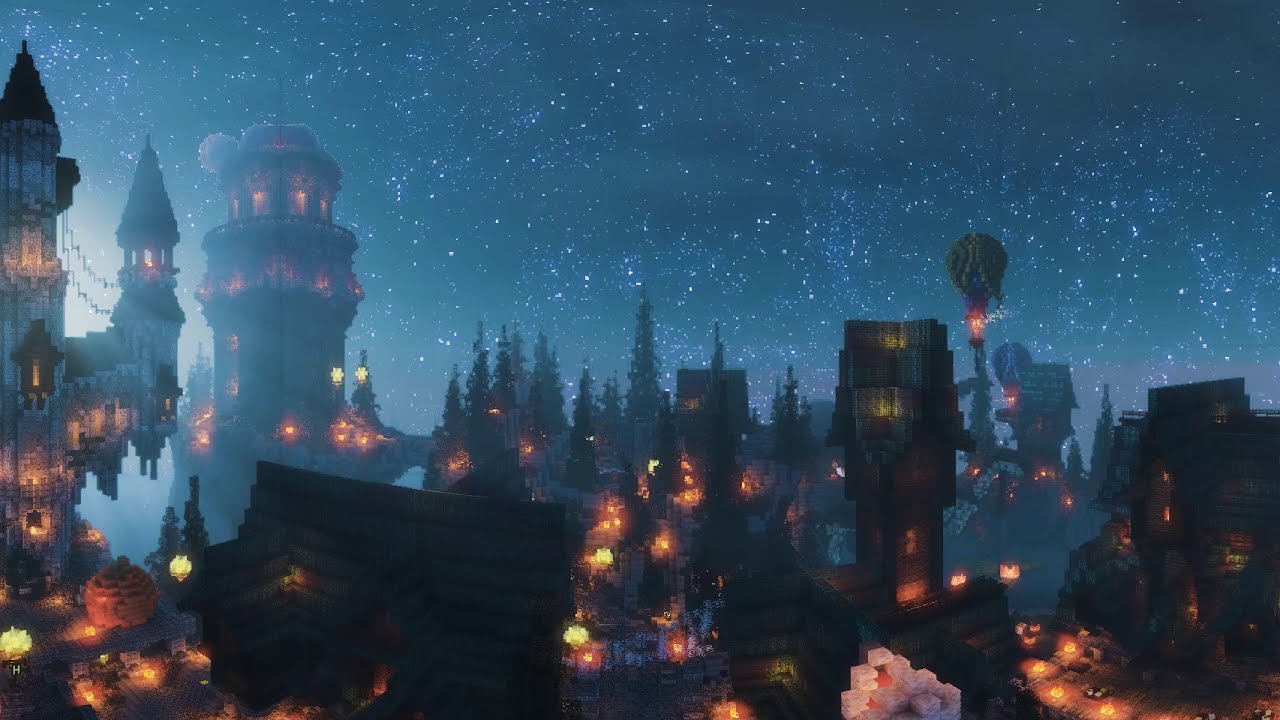This is a horizontally aligned, computer-generated image resembling a high-fantasy, magical scene, reminiscent of a fairy tale or a mystical Minecraft world. The image features a medieval-inspired village in the foreground, illuminated by numerous lanterns that cast a warm yellow-orange glow across the scene. On the left side, there is a tall, stone tower with two turrets and conical or dome-shaped tops, standing as the tallest structure in the village. In the background, additional towers and shorter buildings can be seen, all contributing to the medieval aesthetic. The village is speckled with tall and small evergreen trees, adding to the enchanting atmosphere. The night sky above is a dark blue, blended with lighter hues, and dotted with countless tiny white stars, enhancing the magical feel of this very detailed, pixelated evening scene.